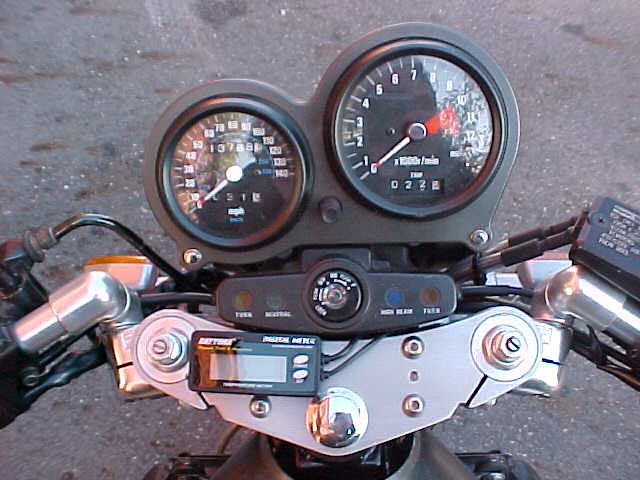A detailed, cleaned-up caption for the image could be:

"An outdoor shot looking down at the control panel dashboard of a motorcycle. We see a circular tachometer on the right and a slightly smaller circular speedometer on the left, both with white indicator dials. The speedometer includes two odometers: one for the total distance traveled and one for the trip distance. The tachometer features a red wedge at the upper end, indicating the danger zone for high RPMs. The handlebars extend on either side of the panel, which also includes several indicator lights, though 'TURN' is the only one legible. Additionally, there is a black rectangular add-on device with an LCD display and two buttons. In the background, the surface appears to be a concrete or packed gravel road."